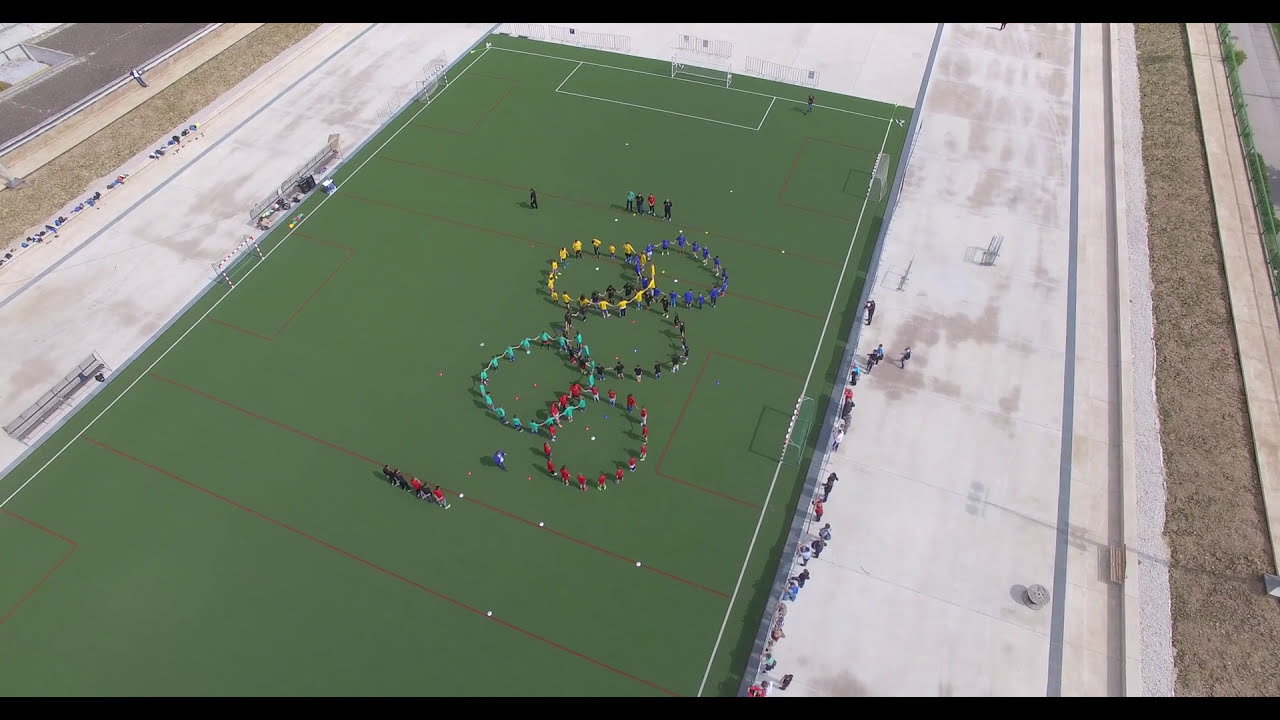The image is an aerial view of a green soccer field, which appears to be taken from a diagonal perspective starting from the lower left-hand corner. The field, a large rectangle, features white and red markings and is bordered by light-colored cement. Surrounding the field are rocky gravel areas and a small fence in the upper right-hand corner, along with a gray roadway in the upper left-hand corner.

In the center of the field, five groups of people form interlocking rings that resemble the Olympic rings. Each group is dressed in different colored shirts: red, green, black, yellow, and blue. From bottom to top, the arrangement of the colors starts with red, followed by green, black in the center, yellow, and blue at the top. Despite some variations in the stated colors, the overall formation mirrors the iconic Olympic symbol.

Additionally, there is a small crowd of spectators along the right edge of the field, although they appear tiny and indistinct from the high vantage point. A thin black bar runs horizontally across the top and bottom of the image, framing the overall scene.